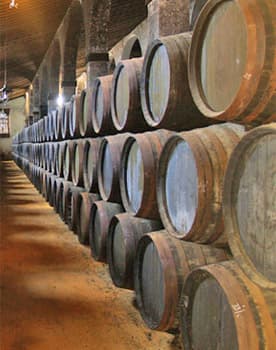The image depicts a long, warehouse-like room, potentially a wine cellar, characterized by a dirt path floor and a series of stone arches on the right side. Along the left wall, rows of barrels are meticulously stacked on top of each other, forming three tiers that extend into the distance. Each row comprises approximately 20 barrels, creating an impression of depth with a worn, rustic aesthetic. The walls are a grayish hue, complementing the dark-colored roof, while the overall setting exudes an aged, historic charm.